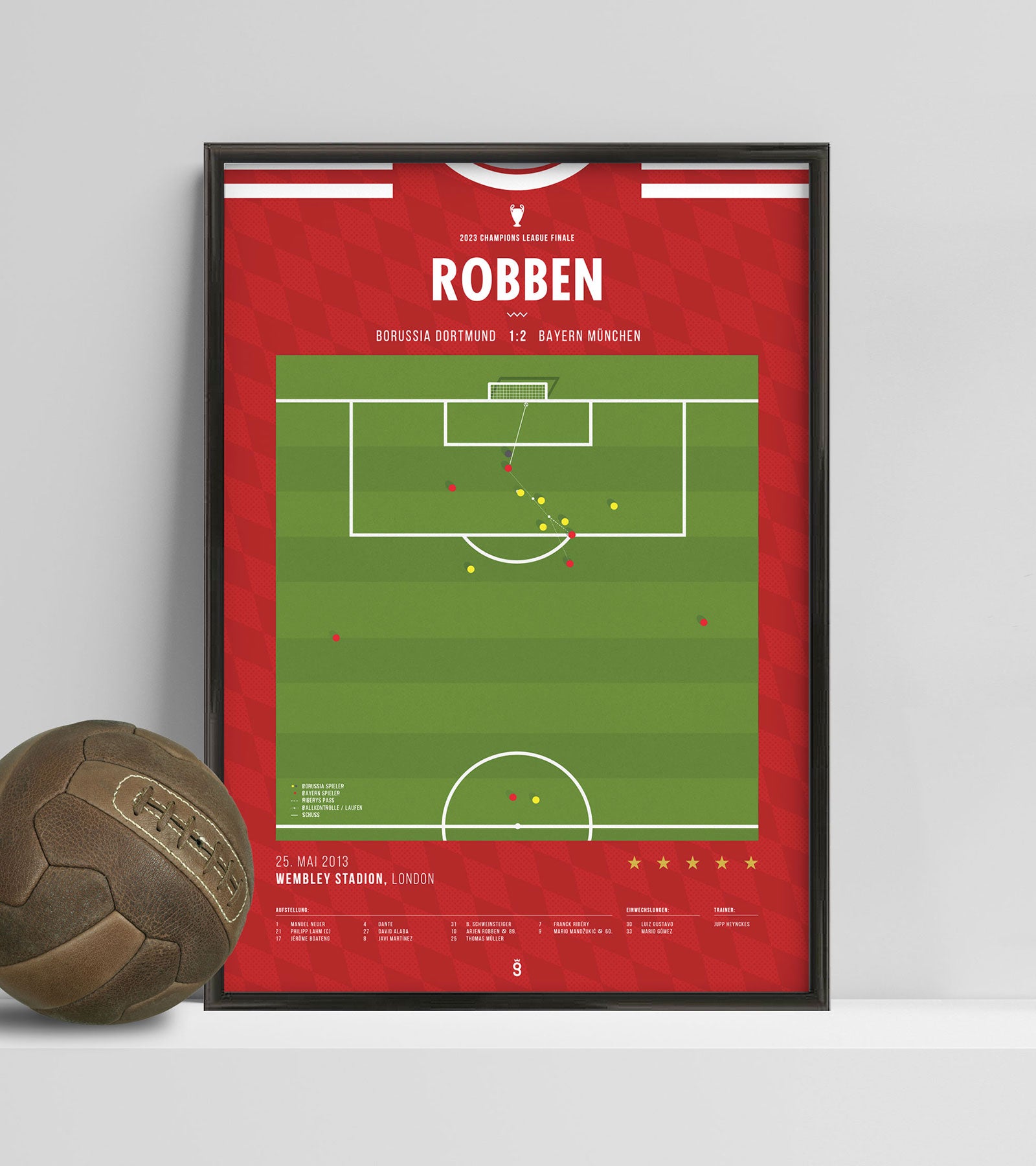The framed poster commemorates the 2013 Champions League Final between Borussia Dortmund and Bayern Munchen, held on May 25, 2013, at Wembley Stadium in London. The poster is framed with a black border and displays a red background with a darker red grid resembling a jersey. At the top, it prominently features "ROBBEN" in white text, marking the key player, and the score "Borussia Dortmund 1 - 2 Bayern Munchen," with the 'u' in Munchen highlighted by two dots. The bottom of the poster notes the date "25 MAI 2013" and the location, with additional details such as a depiction of a football field showing the player positions in yellow and red dots and the trajectory of the winning goal. A dark brownish-green soccer ball with laces, possibly an antique, is displayed next to the poster, which all sits against an off-white wall. The details also include emphatically the five stars at the bottom right corner, symbolizing the grandeur of the event.